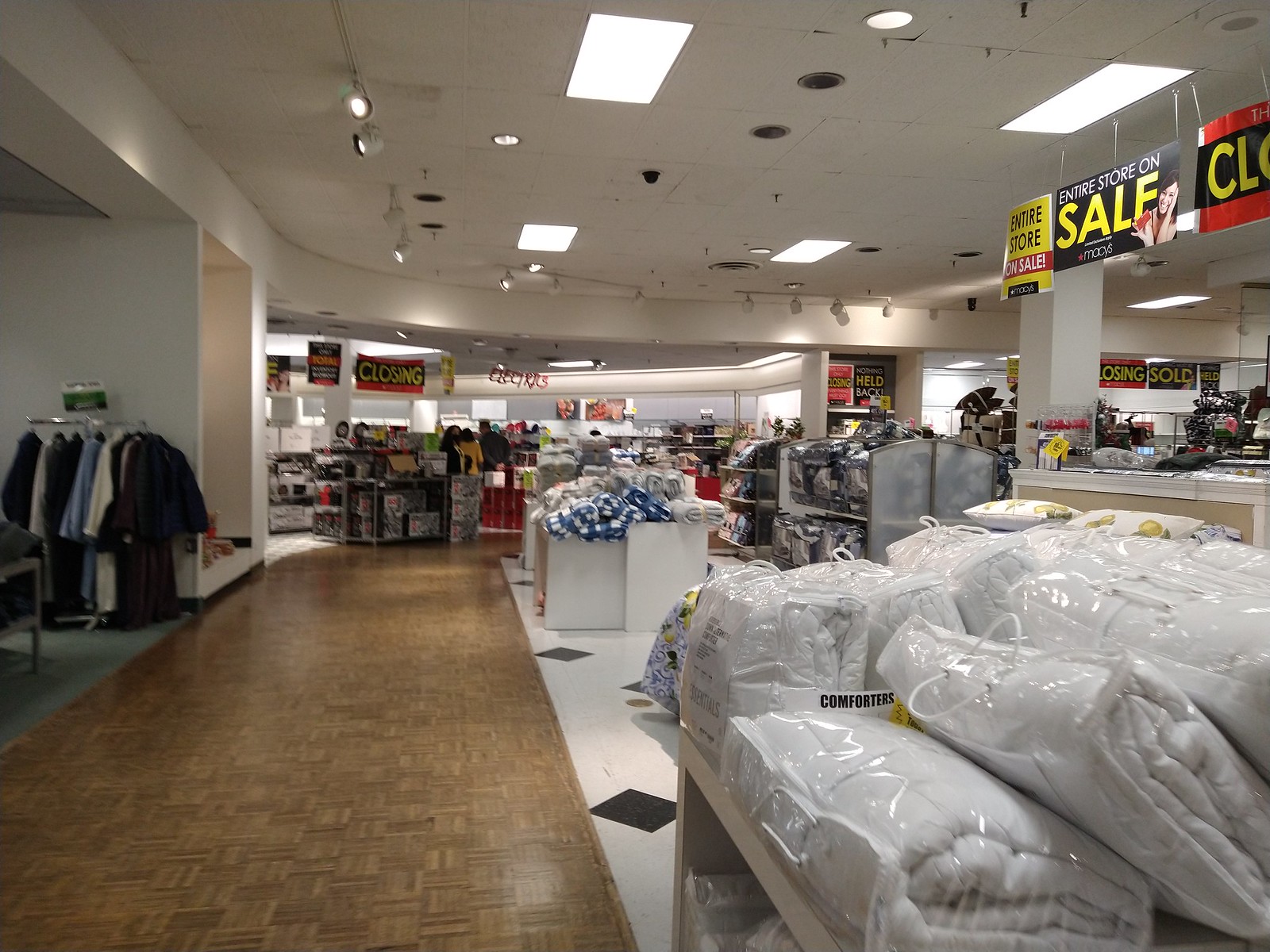This image captures a forlorn scene from a department store in the process of closing down. In the bedding department, a table display prominently features a selection of all-white comforters, with additional shelves underneath housing more bedding items. To the left of the display, you can see a section of clothing. The floor consists of white tiles intricately patterned with small alternating brown diamonds. The walkway features a woodgrain design reminiscent of the parquet flooring typical of Boston Square Garden, adding a touch of elegance. The entire store is dimly lit in the standard, non-glaring manner typical of department stores, suggesting a sense of normalcy amid the closure chaos. Across the store, various items are marked down, signaling the unmistakable signs of liquidation. Racks and merchandise fill the background, yet the specific details are indistinct, adding to the overall atmosphere of a store in its final days. It’s a poignant scene of a once-thriving retail space now facing its imminent end.